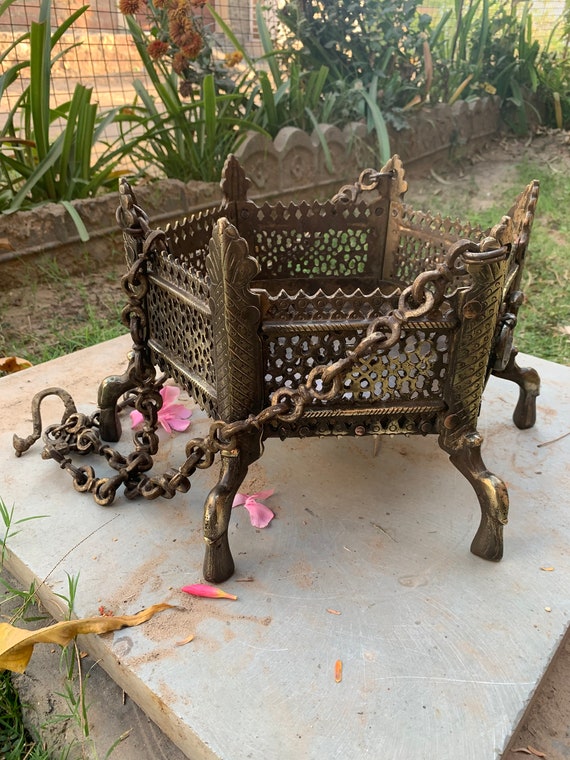The image depicts an outdoor garden scene captured during the golden hour, either at sunrise or sunset. On the left side of the image, there’s a mesh fence partially obscured by various plants and stones, suggesting a cozy, enclosed garden area. The focal point of the image is a square cement slab on which sits a decorative, six-sided metal container. This container appears to be made of aged copper or iron, exhibiting a golden or bronze patina with some rusting. The container, which might function as a fire pit or a decorative garden feature, is intricate and has legs that lift it off the ground. It is also adorned with a heavy chain secured to three of its sides, potentially for hanging. The background shows a decorative brick lining and more plant life, enhancing the image’s garden setting.